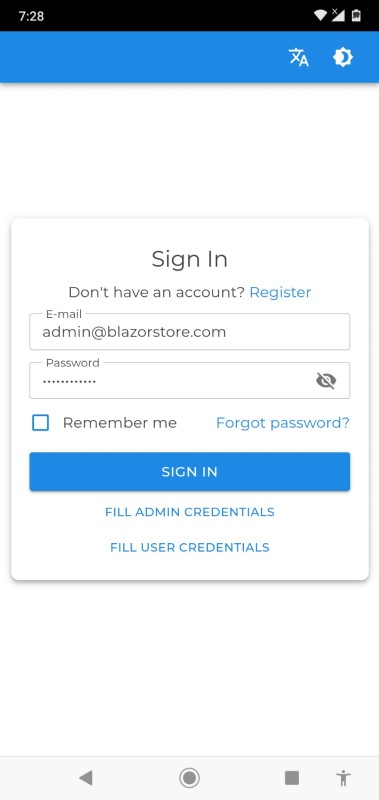The image depicts a sign-in screen on a smartphone. At the top, there's a black status bar which includes the time "7:28," along with indicators for Wi-Fi, signal strength, and a battery meter showing approximately 30% charge. Directly below, a light blue banner spans the width of the screen, featuring the Google Translate icon with a symbol resembling a Korean or Japanese character inside the letter 'A'. Next to this icon, there are two smaller icons representing a sun and a moon, likely for toggling between light and dark modes.

Further down, there is a prominent white field housing the sign-in area. At the top of this section is a floating pop-up that reads "Sign In." Below this, a message states, "Don't have an account? Register," with 'Register' highlighted as a clickable blue link.

The main sign-in form contains two input fields labeled 'Email' and 'Password', outlined with thin gray lines. In the email field, the address "admin@BlazorStore.com" has been entered. The password field displays 10 masked characters, represented by dots, with an 'eye' icon slashed through, indicating the password is hidden. Below these fields, there is a "Remember Me" checkbox, which is currently unchecked, and a "Forgot Password?" link in blue positioned to the right.

At the bottom, a large blue "Sign In" button with white text encourages users to proceed. Beneath this button are two additional blue text links in all caps: "FILL ADMIN CREDENTIALS" and "FILL USER CREDENTIALS". This sign-in section is highlighted with a faint gray drop shadow, separating it visually from the rest of the screen.